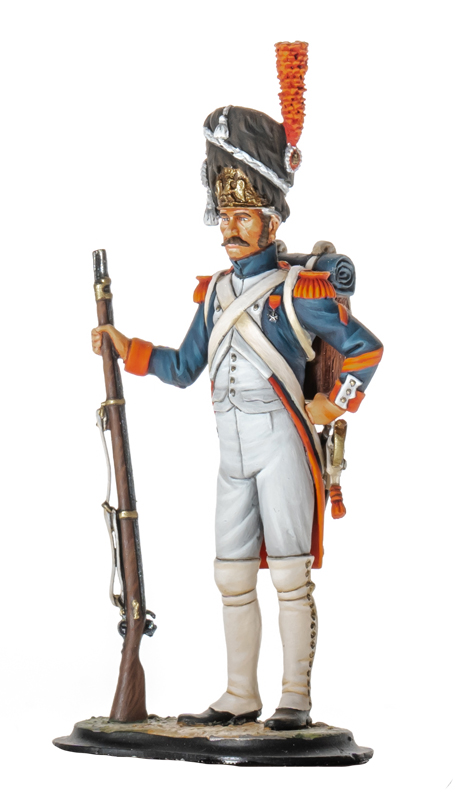This is a color photograph of a highly detailed miniature figurine depicting an older era soldier. The figurine stands on an oval, dark-colored pedestal and is facing to the left, exuding a very serious and somber expression. The soldier is dark olive-skinned with a distinct mustache and long sideburns. He is adorned in a striking military uniform, featuring a tall black hat with a gold emblem and a tall, feathery red decoration on the right side. His blue jacket boasts orange accents on the shoulders and sleeves and overlays a white vest and pants. The soldier's white boots have covers that extend just over his knees, decorated with buttons up the sides. The figure's right arm is bent at the elbow, holding a long rifle with gold accents close to his face, while his left hand rests on his hip. Attached to his back by cross straps, he carries a knapsack with a rolled-up sleeping pad visible. The detailed attire and posture suggest the soldier is prepared for battle, encapsulating a moment frozen in time.